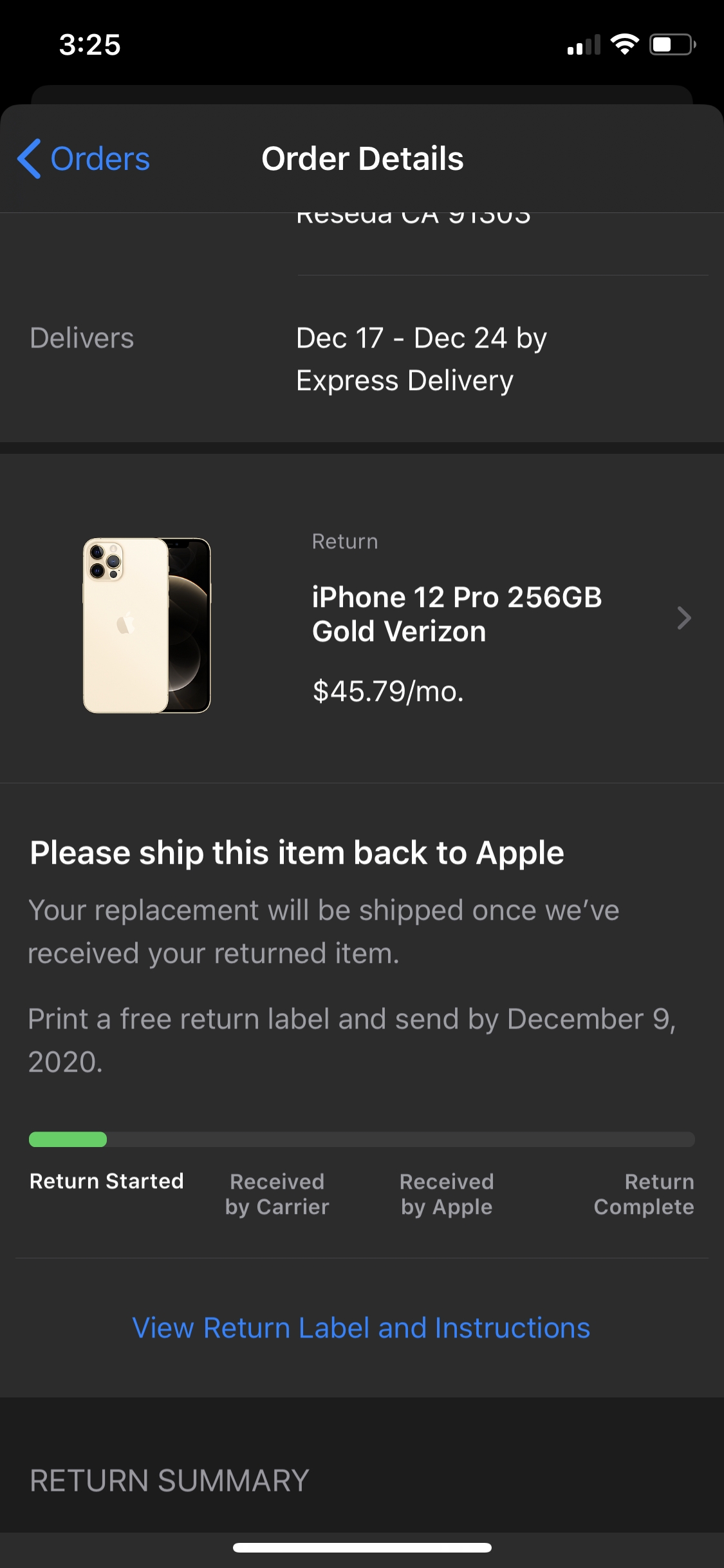**Detailed Caption:**

This screenshot displays an order page with a dark gray header bar spanning the entire width of the page. On this header, "Order Details" is prominently present. To the left of this title, there is a blue "Orders" button accompanied by a back arrow pointing backward.

Beneath this header, the page is divided into two primary sections. On the left, there is a delivery status column indicating "Delivers" followed by concise details on the right which state the express delivery timeframe from December 17th through December 24th.

Further down, a visual of an iPhone is located on the left side of the screen, while on the right, text specifies "Return iPhone 12 Pro 256GB Gold Version" priced at $45.79 per month. Immediately below is an instruction note asking the user to ship the item back to Apple, with a confirmation that the replacement will be dispatched upon receipt of the returned item.

At the bottom of the content area, there's a progress bar delineating four distinct stages of the return process: "Return Started," "Received by Carrier," "Received by Apple," and "Return Complete." This bar visually tracks the progression of the return status.